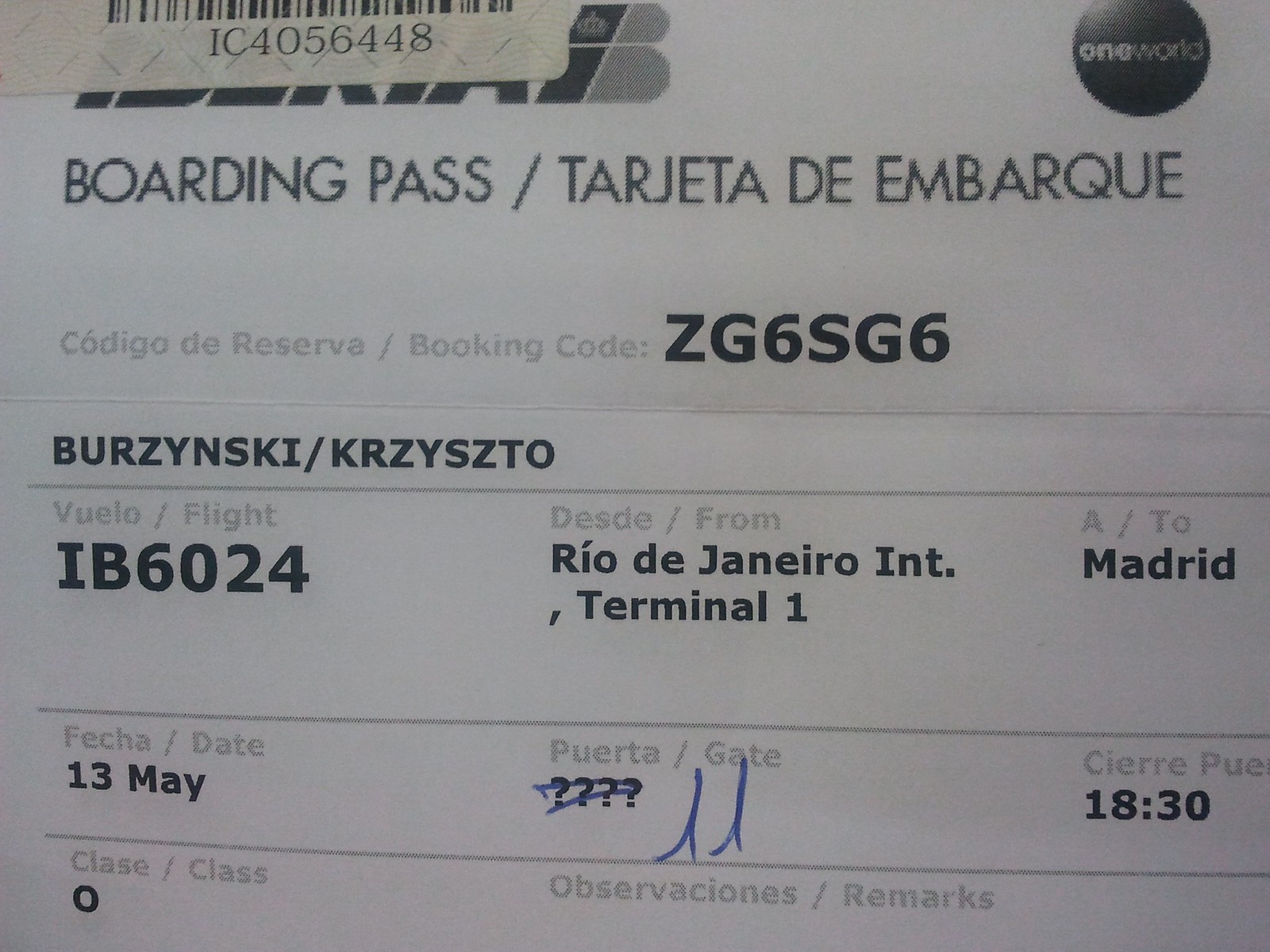The image is a detailed photograph of a boarding pass for an airplane. In the upper left, a barcode is visible with the number IC4056448 beneath it, likely indicating a luggage tag adhered to the boarding pass. Directly below, the text "boarding pass / tarjeta de embarque" is displayed, followed by the booking code "código de reserva / booking code ZG6SG6". In the upper right corner, there is the 'One World' logo encircled by a black ring. The passenger name listed is Brzezinski / Crescisto. The flight information shows flight number IB6024, departing from Rio de Janeiro International Terminal 1 and heading to Madrid. The date of departure is 13 May, and the boarding gate is marked with a handwritten correction in blue ink, indicating gate 11. The boarding pass also notes the flight time as 18:30 and the class of service as O.